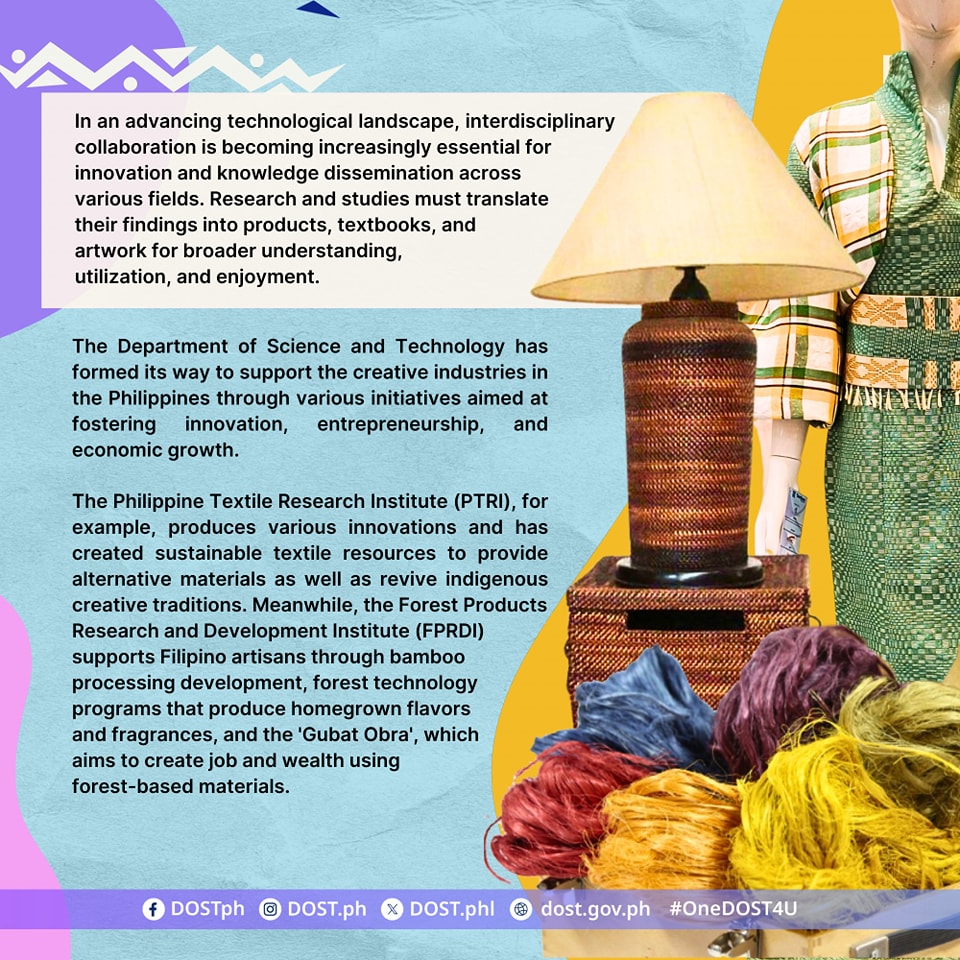The image features an informative banner set against a blue background with a mix of black text and multiple colors. The text emphasizes the importance of interdisciplinary collaboration in today's advancing technological landscape, highlighting its necessity for innovation and the dissemination of knowledge across various fields. It underscores the need for research and studies to be translated into products, textbooks, and artwork for broader understanding, utilization, and enjoyment. To the right of the banner, there's an ornamental lamp with a white shade sitting on a wicker basket. Below the lamp, a small bucket filled with yarn is visible. Beside the lamp stands a mannequin wearing a green apron over a green, white, and yellow patterned shirt. At the bottom of the banner, various social media icons, including links to Facebook and Instagram, are displayed.